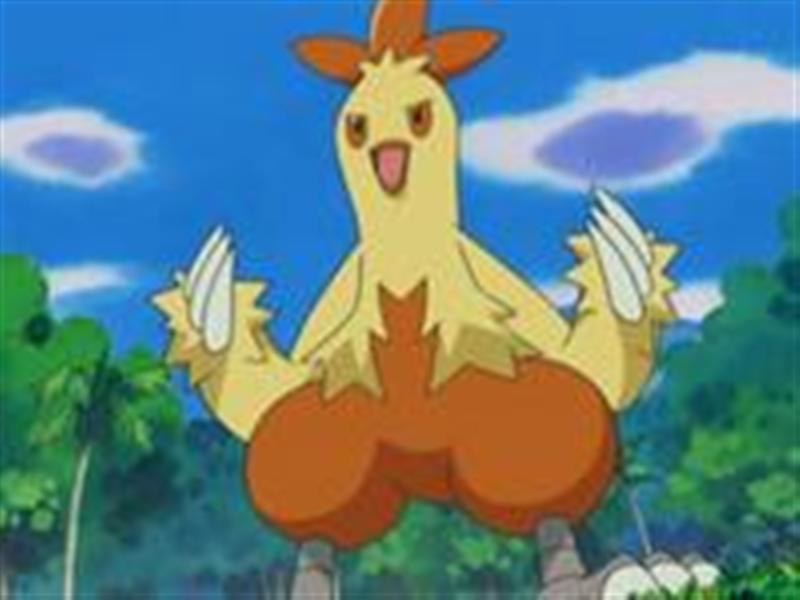The image depicts a cartoon-like Pokémon character resembling a chicken, standing in a defensive or attack stance in a forest clearing. The Pokémon has two grey legs with talon-like feet and talon-like fingers. Its upper body is light yellow while the lower body is dark yellow, and it has a beak, two eyes, and an open mouth, indicating action or speech. The background features green trees, a blue sky, and white clouds, suggesting an outdoor setting during an action sequence from a television show.